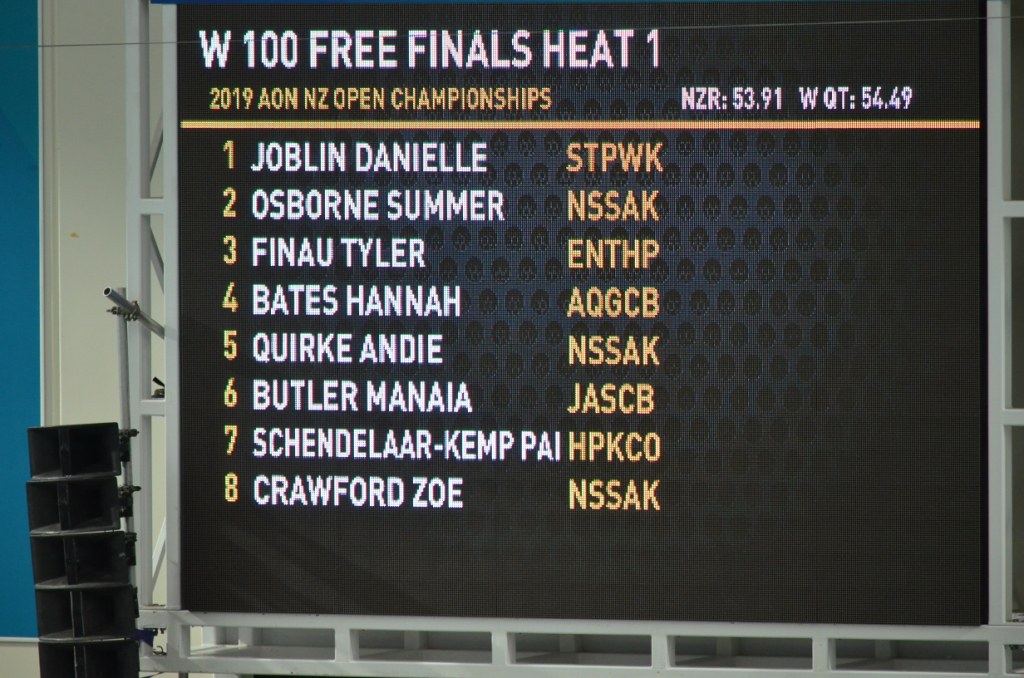The image depicts an electronic scoreboard at a swimming event, specifically for the Women's 100m Freestyle Finals Heat 1. The scoreboard, set against a black background, features white text at the top stating "W100 Free Finals Heat 1." Beneath this, bold yellow text reads "2019 Aon NZ Open Championships." To the right, in white lettering, "NZR: 53.91, WQT: 54.49" is displayed, indicating the New Zealand Record and the qualifying time, respectively. Below, a yellow-orange line stretches horizontally across the screen, segmenting the display. The lower portion lists the names and teams of the eight participants: 1. Joblin Danielle (STPWK), 2. Osborne Summer (NSSAK), 3. Fino Tyler (ENTHP), 4. Bates Hania (AQGCB), 5. Quirk Andy (NSSAK), 6. Butler Mania (JASCB), 7. Chandelar Kempai (HPKCO), and 8. Crawford Zoe (NSSAK). The names are aligned vertically on the left, with their team affiliations in yellow to the right. The scoreboard itself is centrally framed within the image, bordered by gray and accompanied by a blue edge running along the left side, and some indistinguishable objects piled in black to the left of the screen.